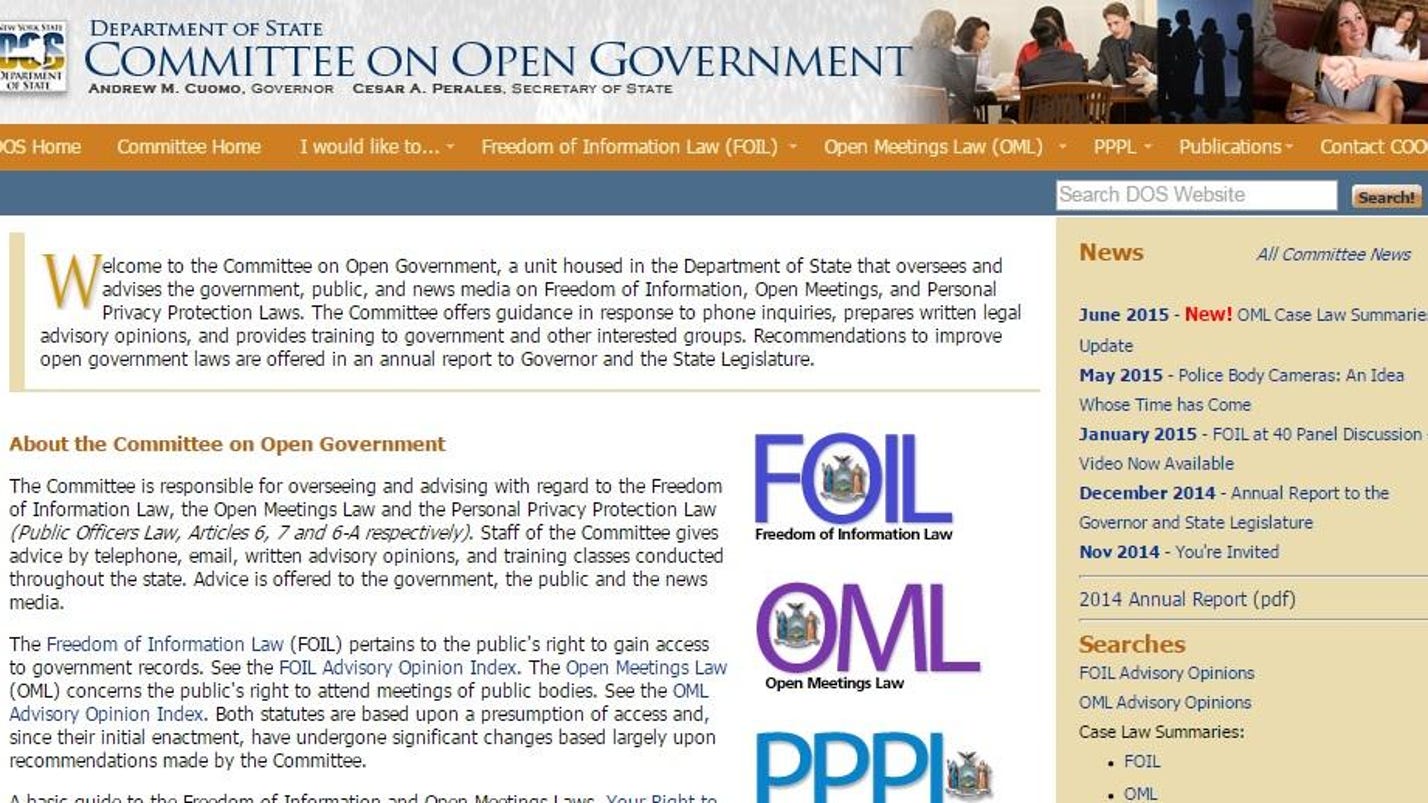The image depicts a webpage of the Department of State, specifically for the Committee on Open Government. At the top of the page, there's an official banner on the upper right-hand corner displaying the text "Department of State Committee on Open Government." Just below the banner, the names "Andrew M. Cuomo, Governor" and "César A. Perales, Secretary of State" are written in black text.

To the right side of the page, there are photographs showing people sitting around a table during a meeting, others standing and conversing in silhouette, and individuals shaking hands in front of a woman. Directly below these images, there are various headers linking to different sections: "Homepage," "Committee Home," "Freedom of Information Law (FOIL)," "Open Meetings Law (OML)," "Public Officers Law (PPL)," "Publications," and "Contact."

Below these sections, there is a block of black text providing a welcoming message and an overview of the committee's functions and additional information about its activities. To the right of this block of text, there's a beige box with blue text that lists dates of important meetings and events. Additionally, there are search fields below this box, allowing users to find more specific information on the site.